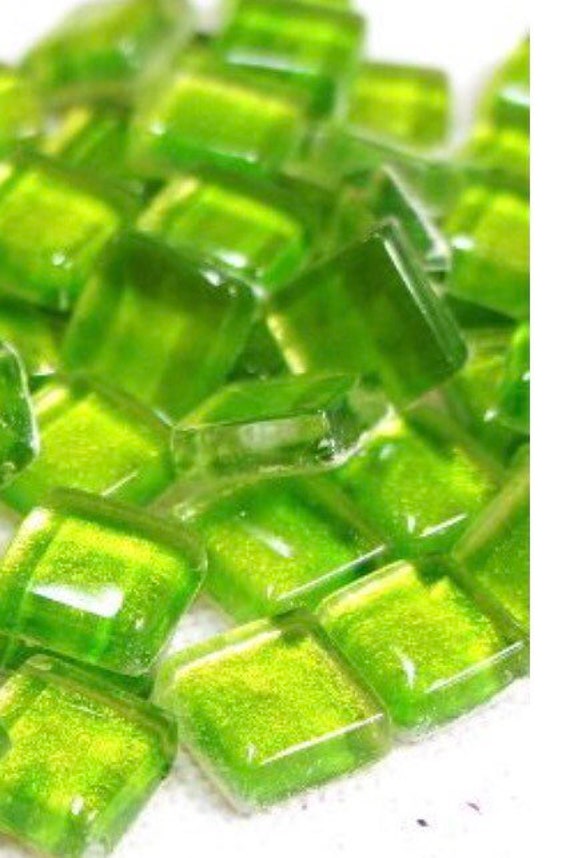This image features a close-up shot of numerous small, lime green candy squares scattered across a clean, white paper towel. The candies are translucent with a glossy shine that reflects the light, creating various shades of green. Most squares measure around three-quarters of an inch, looking smooth and perfect for sucking rather than chewing, suggesting a texture similar to Jolly Ranchers or miniature ice cubes. The white paper towel background, complete with visible fibers and occasional black spots, enhances the clarity of the candies' outlines. With around 40 to 100 pieces present, the candies are layered and bunched together, appearing ready to be enjoyed by someone.